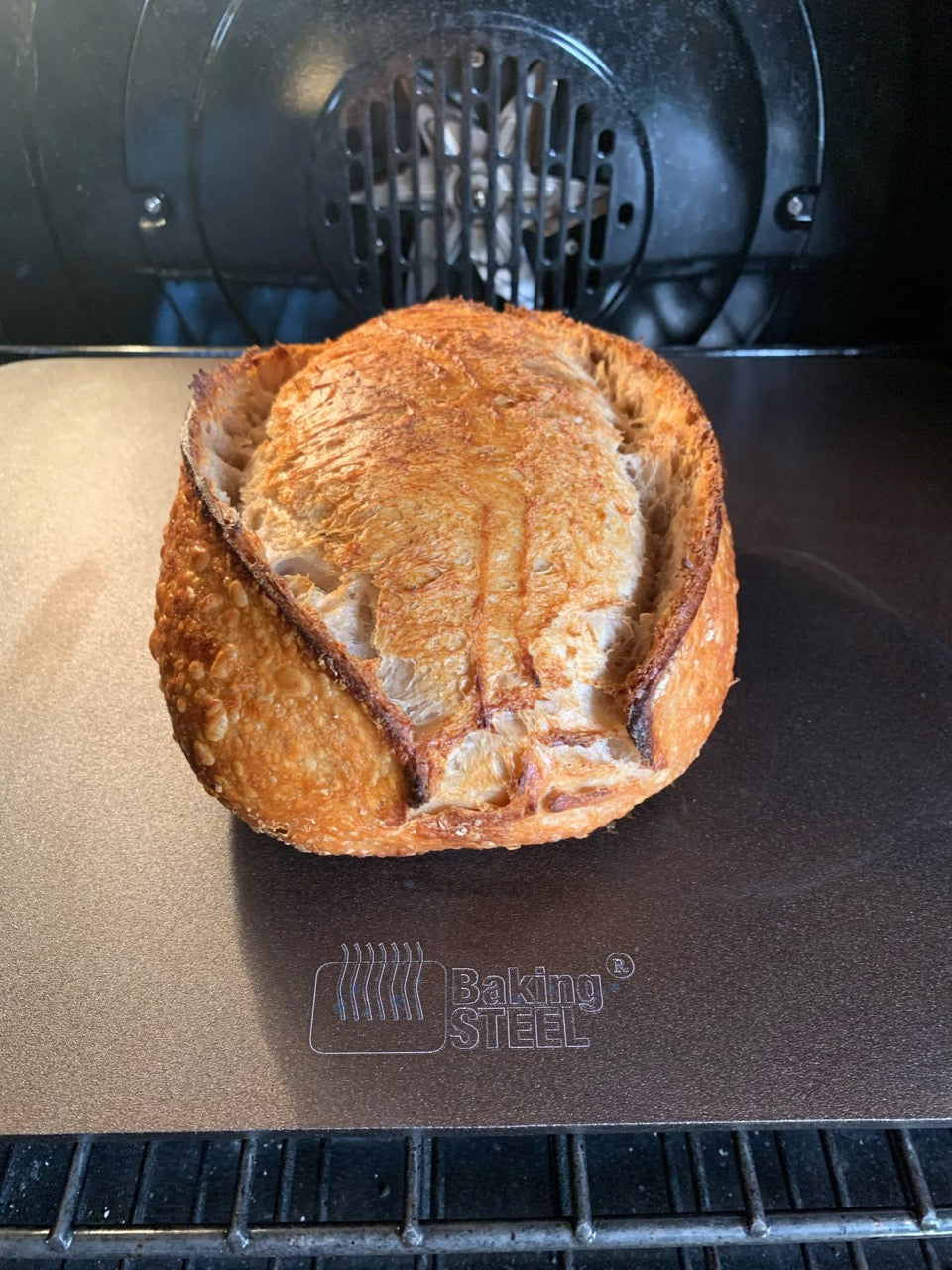The image features a close-up indoor color photograph of a freshly baked loaf of bread in a convection oven. The bread, distinctly risen and oval-shaped, has a hard, crusty surface that has split open at the top, revealing a rustic texture. It sits on a pristine, gray-speckled baking steel sheet, embossed with the "Baking Steel" logo and trademarked at Snotes, depicted as a flat piece of steel with heat wave lines radiating from it. The backdrop reveals a clean, modern oven with a round fan housed within a grate, indicating its use of convection for even baking. The oven's interior is illuminated from the upper left corner, casting the right side of the bread in shadow. This photograph not only captures the artisanal quality of the baked bread but also subtly emphasizes the state-of-the-art baking equipment used, underscoring the efficiency and cleanliness of the baking process.